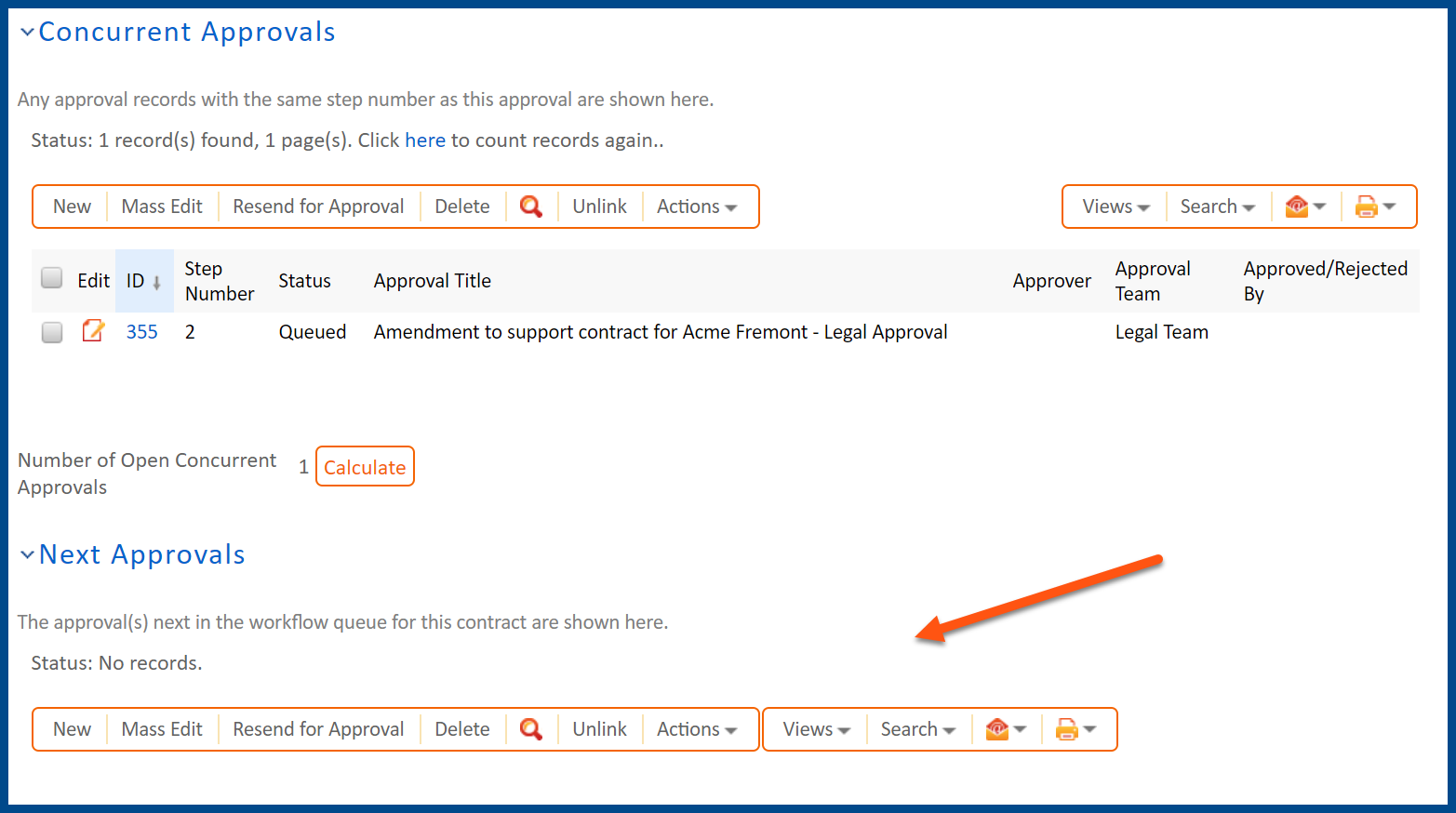This image is a meticulously cropped and edited screenshot, featuring a desaturated blue border and an orange arrow pointing towards the "Next Approvals" section at the bottom. The screenshot captures two expanded drop-down sections: "Concurrent Approvals" and "Next Approvals."

The "Next Approvals" section is highlighted with an orange arrow directing attention specifically to its title. Under "Next Approvals," there is a description that reads: "The approvals next in the workflow queue for this contract are shown here." The status beneath it indicates "No records available."

Below the status, there are two outlined rows of action options. The first row features several side-by-side options: "New," "Mass Edit," "Resend for Approval," "Delete," a search icon, "Unlink," and a drop-down menu labeled "Actions." The second row offers additional side-by-side drop-down menus for "Views," "Search," a mail icon, and a print icon.

Above this, the "Concurrent Approvals" section is visible, showcasing similar rows of action options. Unlike the "Next Approvals" section, the "Concurrent Approvals" section is populated with an approval, providing further context and details for the user.